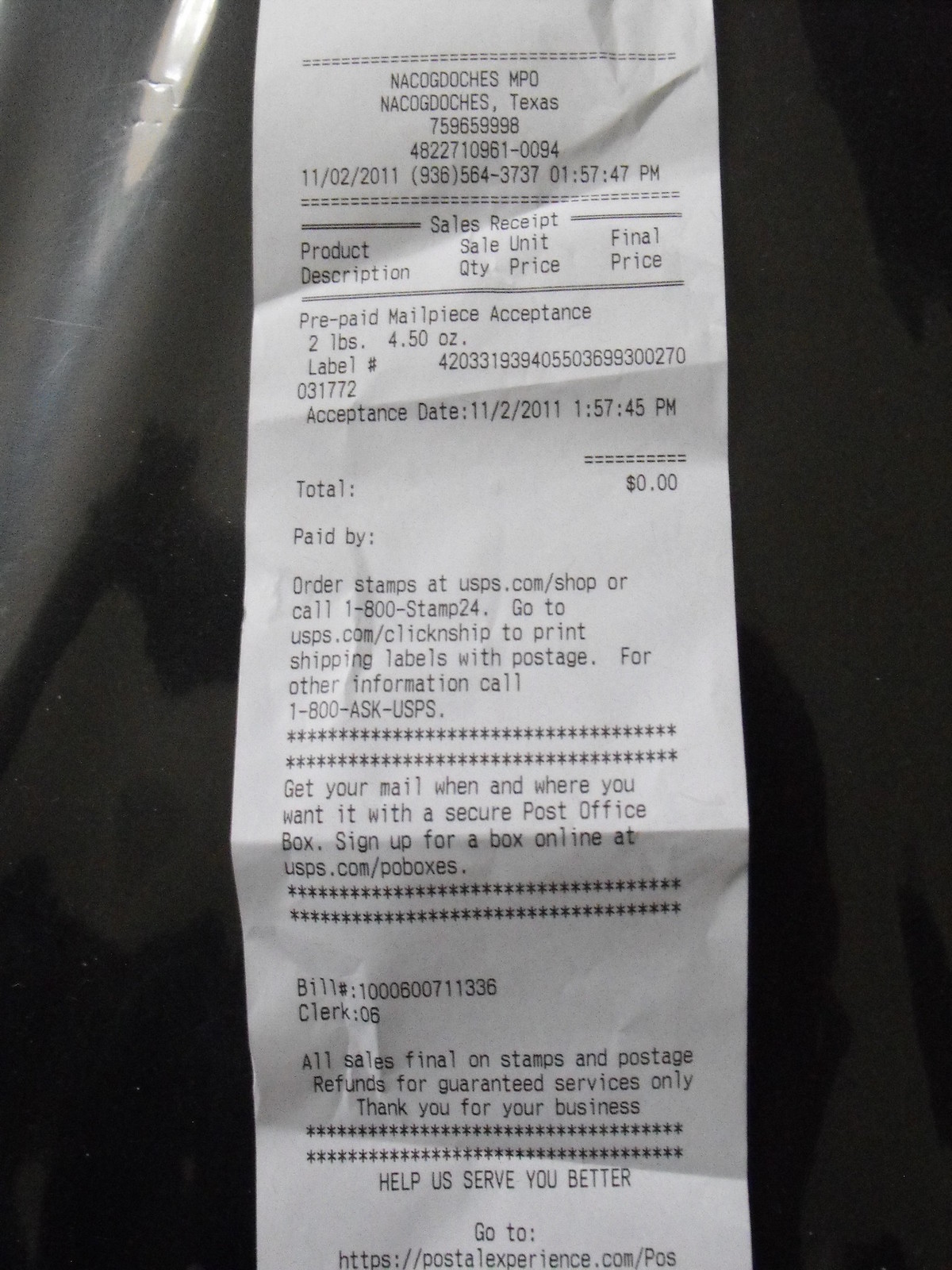This black-and-white photograph features a vertically positioned, long rectangular receipt from the post office in Nacogdoches, Texas, dated November 2, 2011, at 1:57 PM. The receipt, labeled “Nacogdoches MPO, Nacogdoches, Texas 759-659-998,” includes a sales entry for a prepaid mail piece acceptance weighing 2 pounds and 4.50 ounces. Despite displaying a total amount of $0, the receipt details further information such as the phone number, 936-564-3737, and prompts to order stamps at USPS.com or by calling 1-800-STAMP24. Additionally, it encourages customer feedback at PostalExperience.com. The photograph captures a light shimmer diagonally in the upper left corner against a darker background on the right, emphasizing the reflective surface beside the receipt.